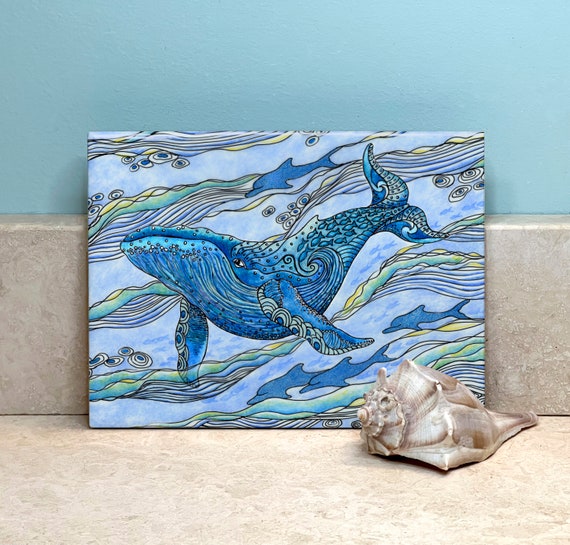This image features a detailed watercolor painting of a happy blue whale, accented with teal, green, yellow, and blue shades, exuding a joyful mood. The whale, marked with intricate designs in light greens and beiges, is the centerpiece of the artwork, surrounded by four similarly colored dolphins. These dolphins appear playful amidst colorful water flow structures, waves, and bubbles. The painting leans against a blue-green wall that suggests a tranquil, aquatic theme. This artistic piece rests on a beige marble-like countertop with a matching short backsplash, potentially in someone's bathroom. Adding to the marine decor, a square conch shell sits in front of the painting, enhancing the oceanic ambiance depicted in the image.